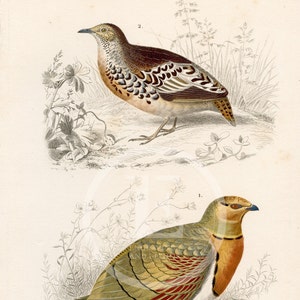This detailed artwork, displayed within a light cream-colored box, features two vividly illustrated birds, likely male and female pheasants, set against a backdrop of intricate line drawings. The upper bird, presumed to be the male, is distinguished by its brownish head, green neck, multicolored wings (brown, green, and yellow), and a brown bib-like chest with a white underside. Its dark beak and speckled, cheetah-like pattern add to its distinctiveness. Pencil or charcoal sketches of foliage, including trees, grasses, and flowers, form the surrounding environment. Below, the presumed female bird is depicted with a toned-down appearance: a dark brown back, speckled brown-and-white underside, light brown bib, and greenish, olive-toned wings with orangish-red highlights. Both birds exhibit dark, striking eyes, with the upper bird’s eye having a reddish hue. A subtle, circular watermark featuring the letter 'E' is superimposed on the artwork, adding a layer of texture.